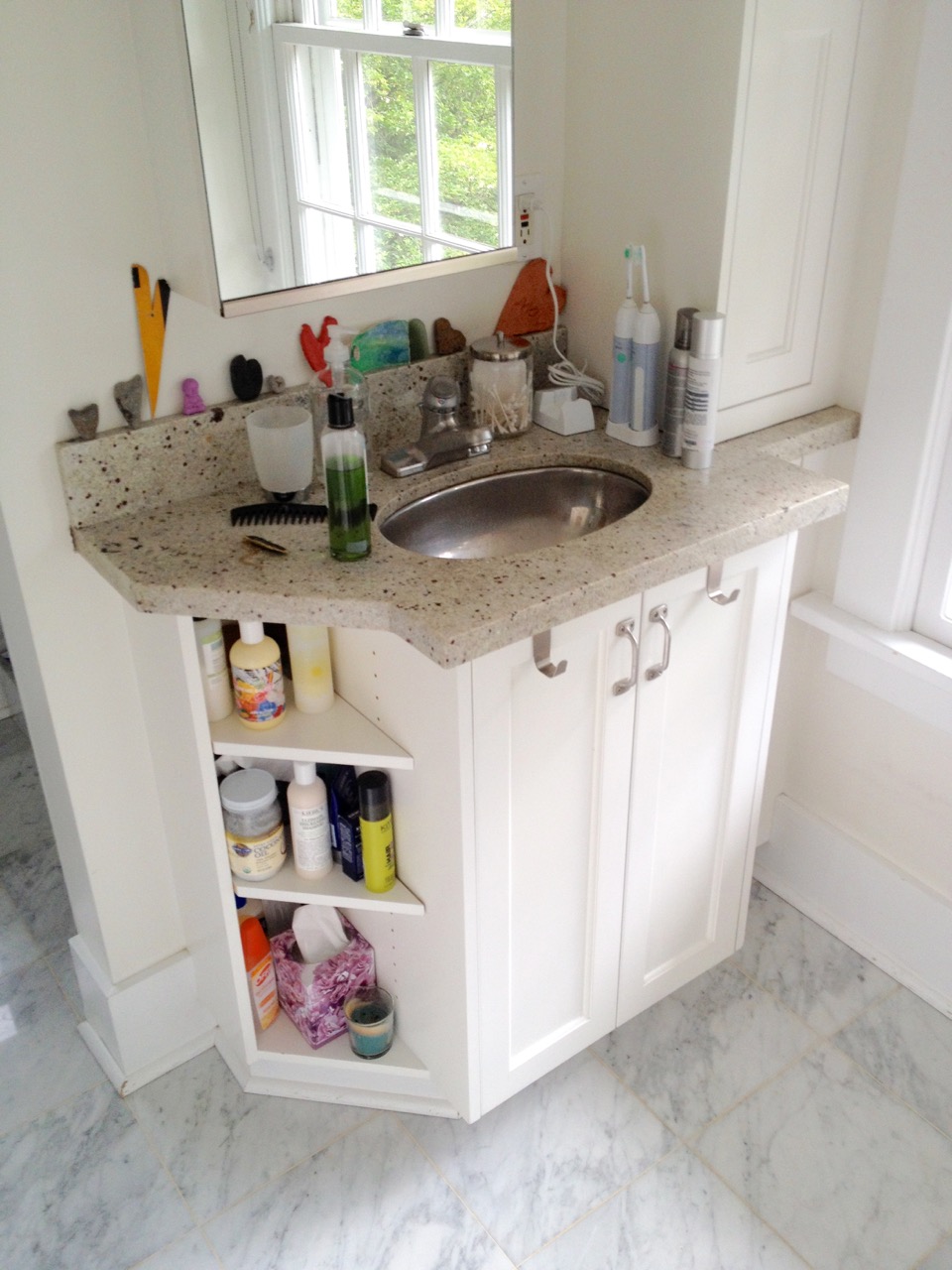This image captures a cozy and well-organized bathroom nook. Central to the frame is a compact vanity unit with built-in white shelves and a beige-brown countertop. The vanity, adorned with silver handles, seamlessly integrates functionality and style. Above the countertop, a mirror reflects the bright light streaming in from a nearby window, through which vibrant green trees are visible, adding a touch of nature to the space.

The shelves within the cabinet are neatly arranged: the top shelf holds various shampoos, the middle shelf is a colorful array of bottles, jars, and sprays, and the bottom shelf houses a tissue box with a pinkish design. On the countertop, a glass for brushing teeth nestles beside a plugged-in electric toothbrush and other personal items, highlighting the efficient use of the small space.

The overall scene is a harmonious blend of practicality and aesthetics, with the colorful bottles adding vibrancy against the backdrop of natural light illuminating the room. The thoughtful arrangement and the glimpse of greenery outside create a bright and inviting atmosphere.